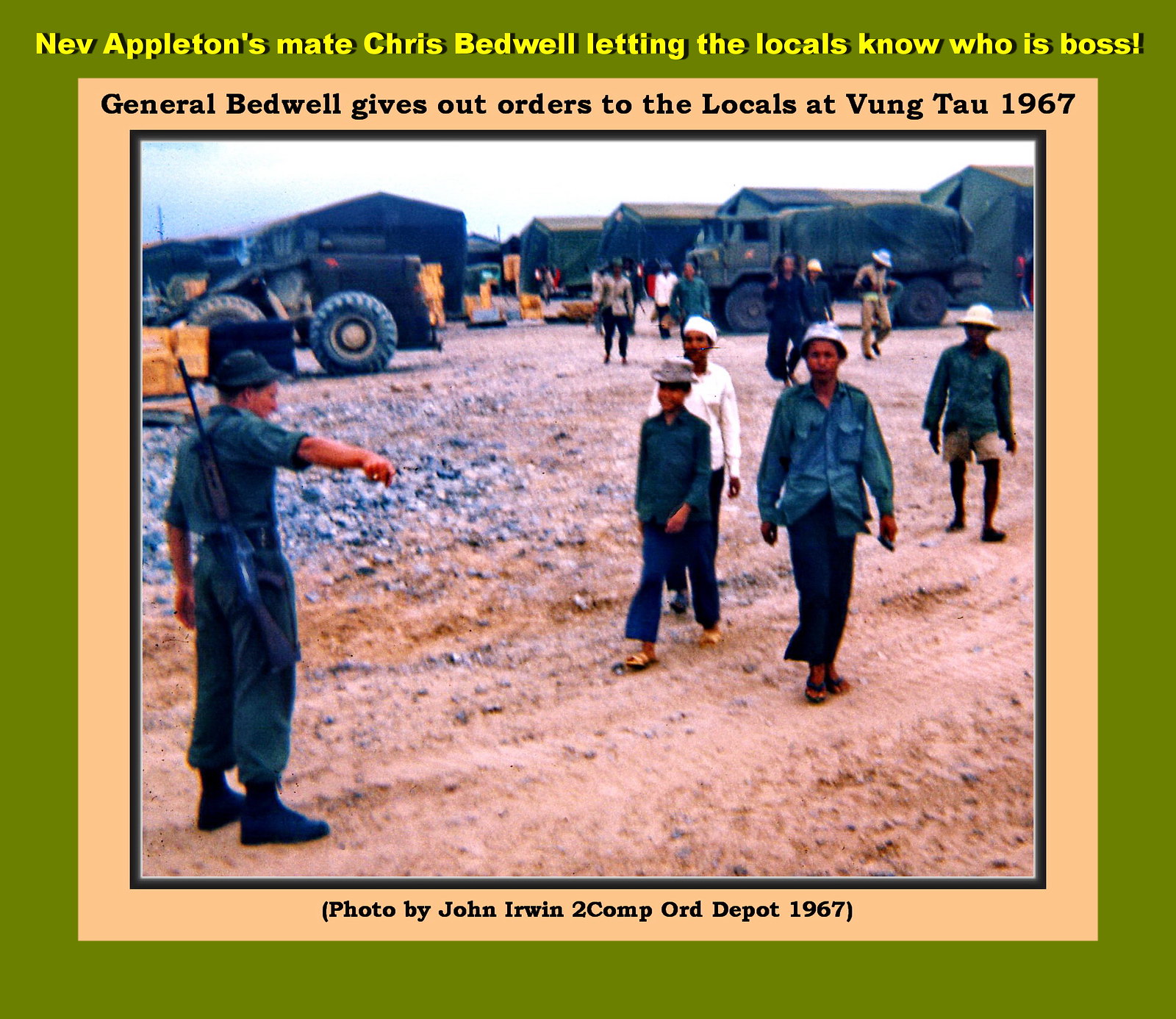The photograph, framed with an orange border followed by a green border, prominently features military activity in a dirt and gravel area devoid of trees or grass. At the top of the green border, text identifies the scene as "Nev Appleton's mate Chris Bedwell letting the locals know who is boss." Within the pink section of the frame, the caption reads: "General Bedwell gives out his orders to the locals at Vung Tau, 1967," and credits the photo to John Irwin, Tukomp, Order Depot 1967.

In the foreground to the left, a soldier in green fatigues, with a gun strapped to his back, gestures directions to a group of Asian men. These men, some wearing white hats and white pants, and others in long-sleeved shirts, blue pants, and sandals, follow his instructions. The group is moving across a terrain of sand and rocks. In the background, large military tents, 20-30 feet long, and resembling barrack tents, dominate the scene. Additionally, there is visible heavy equipment, including bulldozers, large trucks carrying supplies, and yellow buckets. This detailed composition captures a moment of interaction and order amidst an active military context during the Vietnam War in 1967.